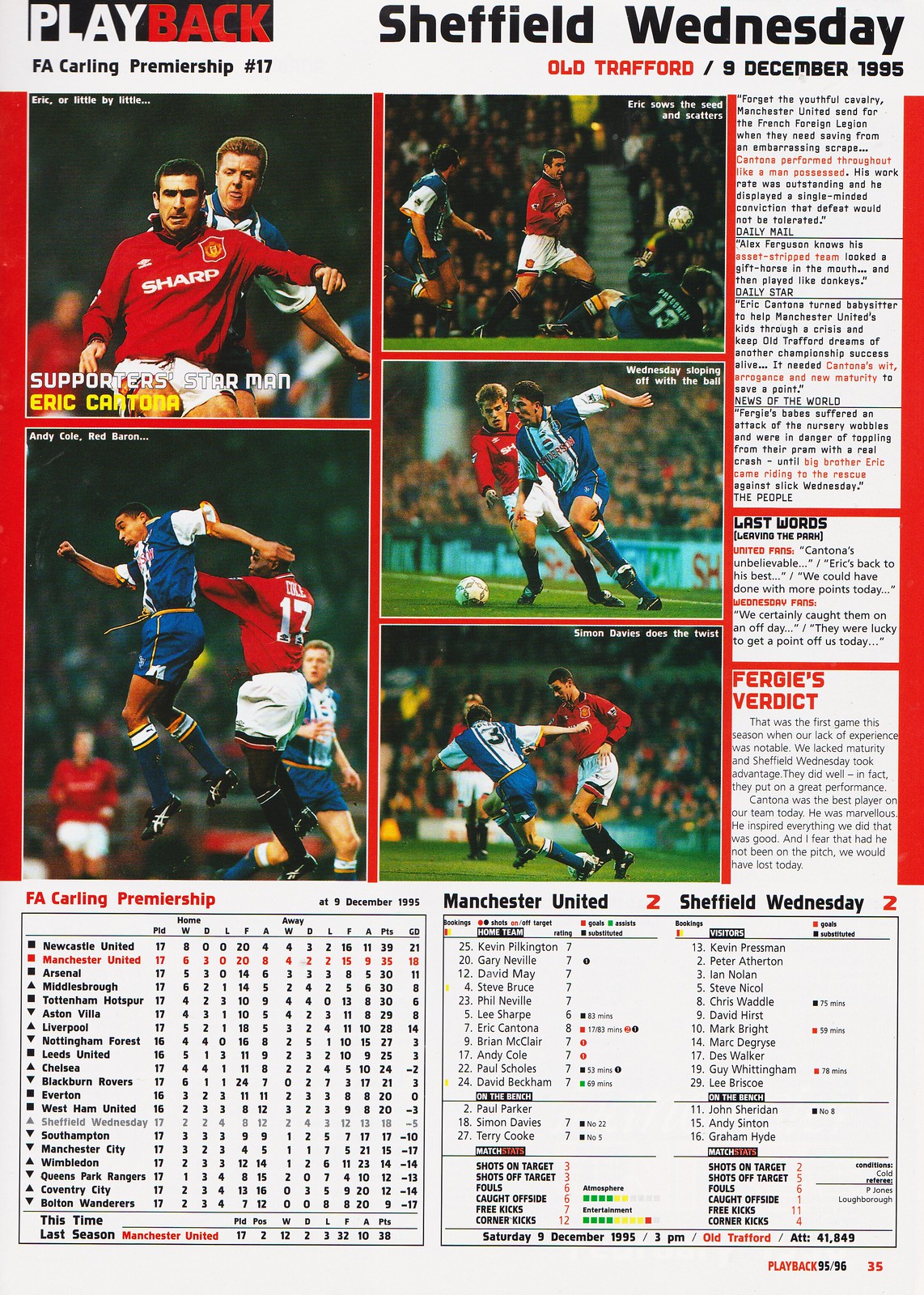This is a scan of page 35 from a football program for a match between Manchester United and Sheffield Wednesday, held at Old Trafford on December 9, 1995, during the F.A. Carling Premiership season 95-96. The page features a grid array of nine color photographs showcasing key moments from the game. Prominently, the top right photo highlights Eric Cantona, labeled as "Supporter Starman," wearing Manchester United's iconic red jersey. The other images capture intense action on the field, with Manchester United players in red and white and Sheffield Wednesday players in blue and white. Above the grid, labels read "Playback," "F.A. Carling Premiership number 17," and "Sheffield Wednesday."

On the right side of the page, there are headers titled "Last Words" and "Fergie's Verdict," featuring quotes and opinions on the game. The bottom section includes standings for the F.A. Carling Premiership on the left, and detailed rosters and stats for Manchester United and Sheffield Wednesday on the right. The page number and the label "Playback 95-96" are noted at the bottom.